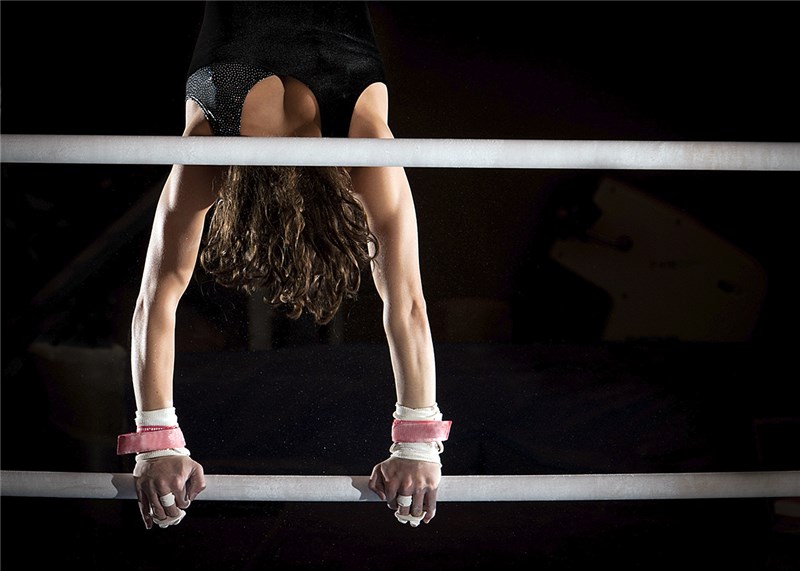A muscular female gymnast is captured mid-routine as she hangs upside down between two horizontal beams. Her medium-length brown hair flows towards the ground, accentuating her inverted position. She's dressed in a black, sparkly tank top, creating a striking contrast against the fully black background. The gymnast's wrists are wrapped in white and reddish gauze, with additional cloth on her middle fingers, likely for extra grip and support. Both bars, which are light gray or off-white, are positioned with one at the top and one at the bottom of the image. Below, her extended body is fully supported by her chalked hands gripping the lower bar, showcasing her impressive strength and control.